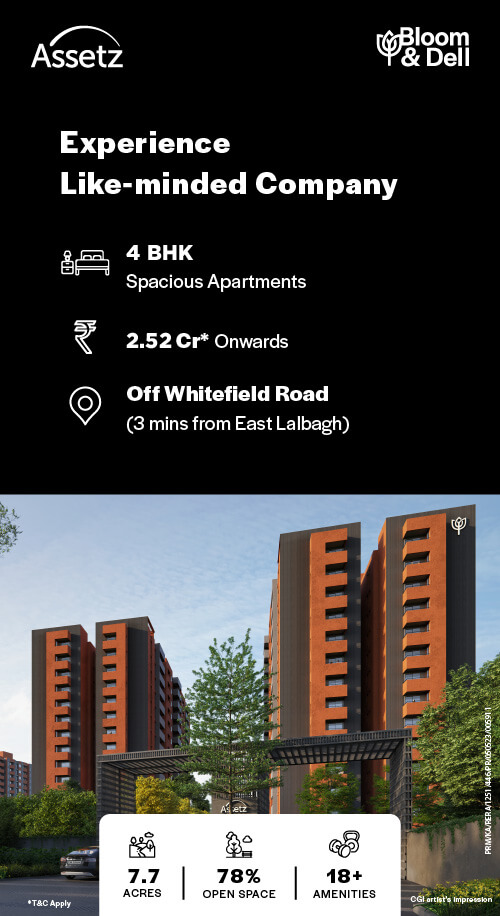*Experience the Charm of Bloom & Dell Residencies: A Detail-rich Insight*

The upper half of this promotional image has a sleek black background. Featured prominently on the left side at the top is the text "ASSETZ" in crisp white letters, crowned by a line arching above it to form a half-circle. On the right side, "Bloom & Dell" is displayed in white, accompanied by a delicate white flower icon to its left. Moving further down, the text "Experience like-minded company" spans two lines in bold white font.

Approximately three lines below that, the layout provides three distinct points, each introduced by an icon. The first point reads "BHK" followed by "Spacious Apartments" below it. The second point portrays the cost: "2.52 CR*" with a note indicating this as the starting price. The third point markets the prime location with "Off Whitefield Road" and specifies its proximity: "(3 MINS from East Lalbagh)."

The bottom half showcases a photograph of the residential buildings. These twin brick structures stand tall and identical, flanking a lush central tree. 

The very bottom features a white rectangular band divided into three columns, each topped with an icon. The first column indicates the expanse of the property: "7.7 acres" in black font. A vertical black line separates this from the next column, which highlights "78% Open Space." Another vertical line divides this from the final column, which notes the "18+ Amenities" available for residents.

---

This curated depiction aims to convey the exclusivity and inviting nature of the Bloom & Dell Residencies with precision and clarity.